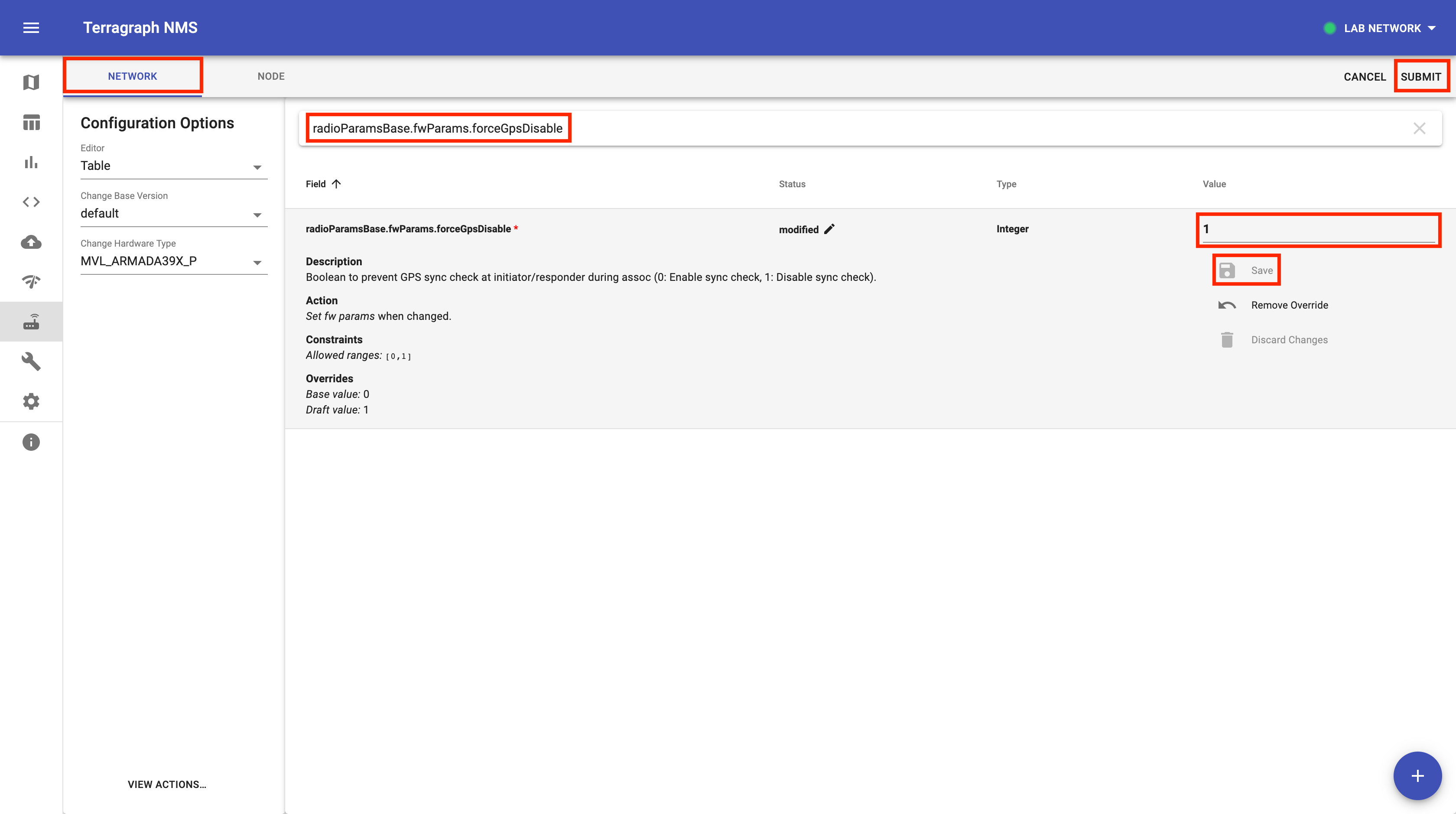The image depicts a webpage or software interface for a program called "Terragraph NMS." At the very top, a long horizontal blue bar spans across the screen, displaying the text "Terragraph NMS" on the left side. On the right side of this bar, "Lab Network" is shown, accompanied by a drop-down menu and a small green indicator.

Directly below the blue bar, the interface is divided into sections. The first section is labeled "Network," highlighted with a red rectangular box. Adjacent to it is a "Node" label. Towards the right side, there are two buttons: "Cancel" and "Submit," the latter also outlined with a red rectangular box.

On the left-hand side of the interface, there are several configuration options followed by three drop-down menus. The first drop-down menu reads "Editor Table." The second one is labeled "Change Base Version Default," and the third is titled "Change Hardware Type," containing a long alphanumeric sequence within it.

Below these menus, there are fields labeled "Field," "Status," "Type," and "Value." At the top, resembling a search bar, there is another red rectangular box containing the text "Radio Params Base.FWParams.ForceGPSDisable." Additionally, there are two more red rectangular boxes with unspecified text located to the right of this search bar.